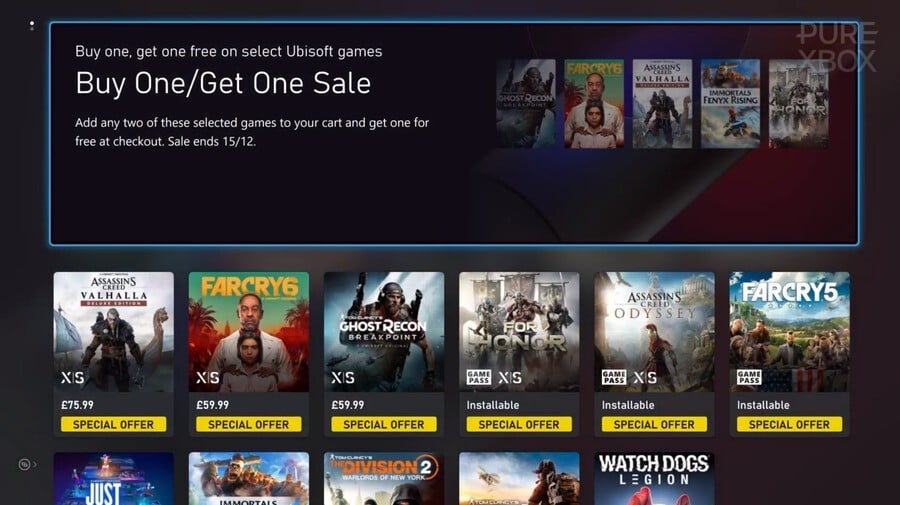The image showcases a screenshot of a website with a black background, set against a white backdrop. At the top of the screenshot, there is a neon blue-lined box containing a promotional message:

**"Buy One, Get One Free on Select Ubisoft Games"**. Beneath this, in larger bold white text, is the caption **"Buy One / Get One Sale"**. Further down in smaller white text, it reads: **"Add any two of these selected games to your cart and get one for free at checkout. Sale ends 15/12."**

Below this promotional box, there is a row of game titles from left to right:

1. **Assassin’s Creed Valhalla** - Highlighted with a **Special Offer** tag in a yellow box.
2. **Far Cry 6** - Featuring an image of an older man and a young man in front of him.
3. **Ghost Recon Breakpoint**.
4. **For Honor**.
5. **Assassin’s Creed Odyssey**.
6. **Far Cry 5** - Marked with a **Game Pass** icon in the lower left corner, along with the notations **"Installable"** and **"Special Offer"**.